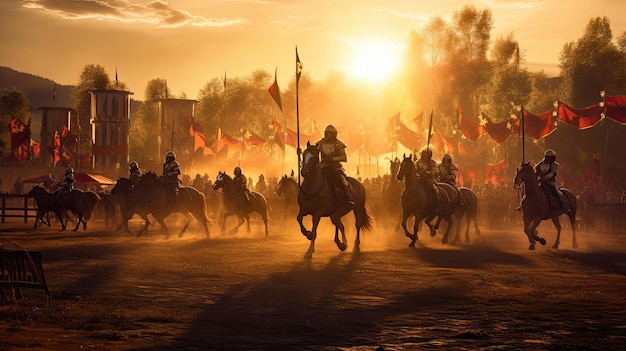This painting, rendered in realistic detail, depicts an army of knights riding into battle. The scene is set on a dark brown ground, upon which several brown horses march forward, each ridden by men clad in full metal armor. These knights are equipped with various weapons and long, tall red flags and banners that flutter in the background. Behind them is a crowd that might either be additional soldiers or onlookers, most of whom also hold red-colored flags. Adding to the complex composition are clusters of green trees and a few buildings located on the left side of the painting. The sky above is bathed in a creamy tan color, illuminated by a brilliant white sun whose rays cast a vivid, bright light onto the ground. The sunlight highlights the knight in the forefront, casting him in silhouette and obscuring details of his face and weaponry, while giving the scene an overall amber and yellow hue that suggests the early morning sunrise, intensifying the sense of an imminent battle.